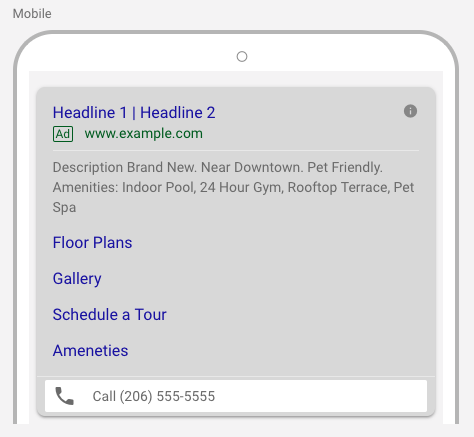A detailed screen capture of the upper half of a mobile app is displayed on a graphic representation of a mobile phone, focusing solely on the top portion of it. In the upper left corner, the screen indicates "mobile" in small text. The background is a light gray shade. Prominently, in the upper left section of the main field, the text "Headline 1" and "Headline 2" are displayed in a light blue font. Directly below this, it reads "Add," followed by a web address "www.example.com" positioned to the right.

A thin white horizontal line separates the header from the body content. Underneath this, in gray font, there is a detailed property description including phrases like "Brand New," "Near Downtown," "Pet Friendly," along with amenities listed: "Indoor Pool," "24 Hour Gym," "Rooftop Terrace," and "Pet Spa." Below these descriptions, navigation options in either purple or light blue font are available, reading "Floor Plans," "Gallery," "Schedule a Tour," and "Amenities."

At the very bottom, there is a white horizontal rectangle, resembling a call-to-action button, which displays a phone number: "Call 206-555-5555." The overall layout appears to be a mockup demonstrating how to configure a mobile app interface, potentially for marketing an Airbnb, apartment complex, or similar property listing platform, showcasing essential details and features prospective users might find appealing.